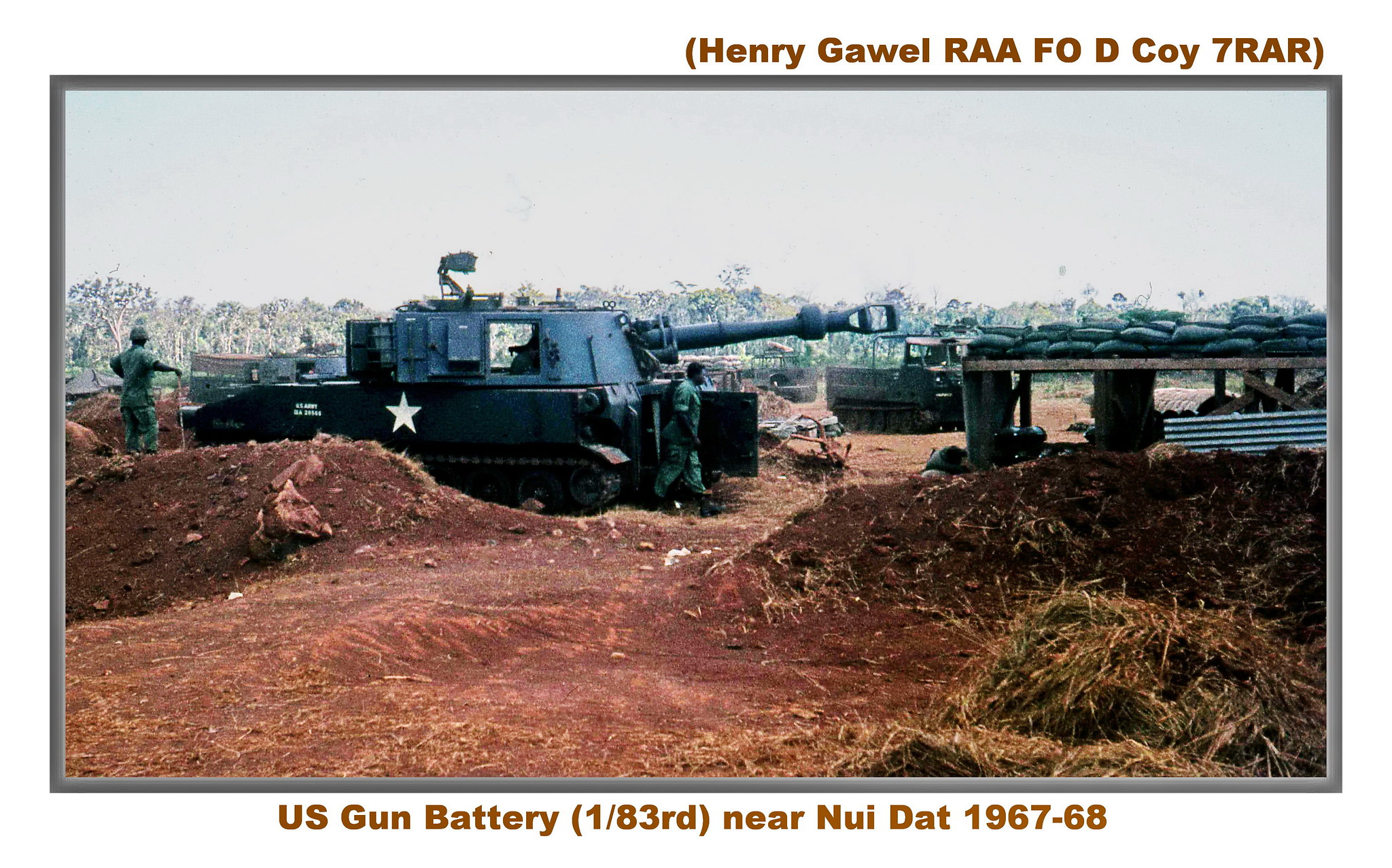In this horizontally aligned, dark gray-bordered photograph, we see a scene from the Vietnam War, specifically depicting the U.S. gun battery of the 1-83rd near Nui Dat during 1967-68. The historical image is topped with brown text reading “Henry Gawal, RAAFOD Coy 7 RAR” and text beneath it that says “U.S. Gun Battery (1-83rd) near Nui Dat, 1967-68.” The central focus of the photograph is an American tank adorned with a white star, with its cannon prominently protruding. In front of the tank, black sandbags are stacked on a raised platform. Two American soldiers are positioned around the tank, one standing behind and one in front. The tank is situated on a field characterized by dirt with scattered mounds and a hint of grass in the lower right corner. The sky above is obscured by a gray haze, which could suggest cloudy weather or smoke, and trees loom indistinctly in the background, shrouded by the same haze. In the background on the right side, a bunker-like structure can be noticed. The overall scene portrays a bleak, war-torn landscape, rich with historical significance.